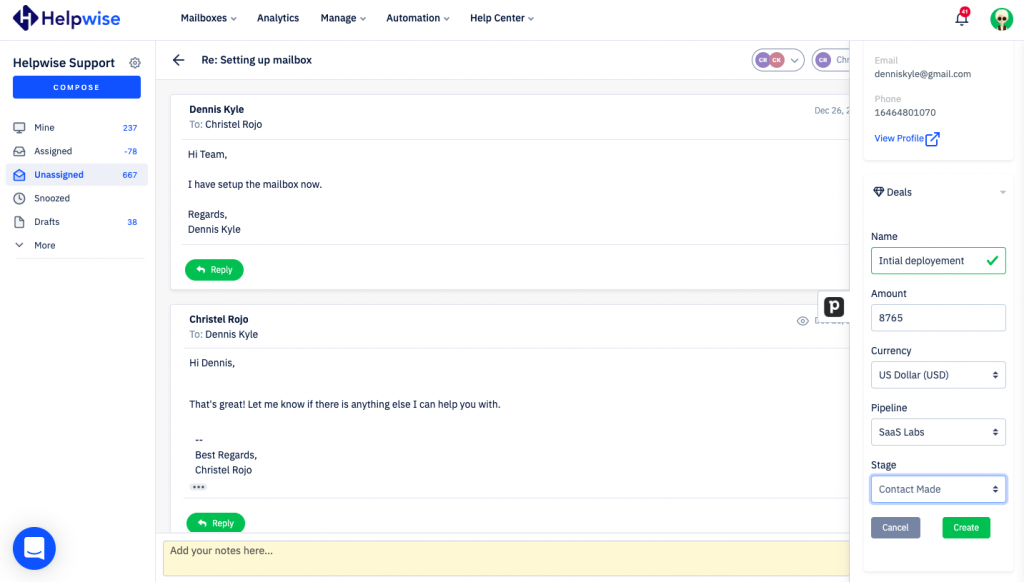**Detailed Caption for HelpWise Webpage Screenshot:**

This image is a screenshot of a HelpWise webpage. The page has a predominantly white background. The HelpWise logo, which is a dark blue diamond shape with a white "H" inside, is prominently displayed. The word "Help" is in dark blue, while "Wise" is in a slightly lighter blue. 

At the top, the navigation bar includes options such as Mailboxes, Analytics, Manage, Automation, and Help Center. 

On the left side, a vertical menu lists options under "HelpWise Support," with a blue button labeled "Compose" in white text. Below this are several categories: "Mine" (237), "Assigned" (78), "Unassigned" (667), "Snoozed," "Drafts" (38), and "More," each accompanied by respective icons.

The main content area features an ongoing email thread. The header reads, "Are You Setting Up Mailbox?" Below, Dennis Kyle emails Christelle Rojo, stating, "Hi, team. I have set up the mailbox now. Regards, Dennis Kyle." There's a green "Reply" button beneath this message. Christelle Rojo's response follows: "Hi, Dennis. That's great. Let me know if there's anything else I can help you with. Best regards, Christelle Rojo," which is also followed by a "Reply" button.

At the bottom of the main area, a yellow-beige box prompts users to "Add Your Notes Here."

On the right-hand side of the screen, there's a notification bell with a red dot. Alongside, there is a green circle icon featuring a person with sunglasses. The contact information for Dennis Kyle is displayed: "Email: DennisKyle@gmail.com, Phone: 1646-480-1070," with a "View Profile" link in blue. 

Below this, a section titled "Deals" shows. Next to it is a small diamond icon. The subsequent fields include:
- **Name:** A green box with the words "Initial Deployment," though "Deployment" seems to be misspelled.
- **Amount:** Listed as "8-7-6-5," with the currency indicated as U.S. Dollars.
- **Pipeline:** Labeled "SAAS Labs."
- **Stage:** A blue box that says "Contact Made."

At the bottom, there are "Cancel" (gray button) and "Create" (green button) options for user actions.